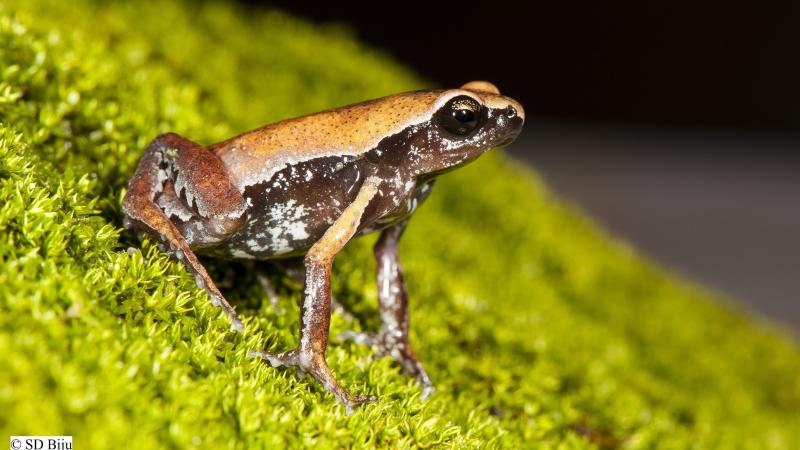The photograph features a small, vividly colored frog perched on very short, light green grass. The frog has a striking orangish hue on its back with a darker underside and big, dark eyes, perfectly capturing its natural elegance. It is positioned with its legs tucked under in the typical frog stance, gazing off to the right. The background is a neutral grey-black, providing contrast to the frog's vibrant coloration. The image appears slightly tilted, with the ground slanting diagonally from the top left to the bottom right. Notably, the bottom left corner bears an artist's signature that reads "S-D-B-I-J-B-I-I-U. Copyright." This detailed photograph emphasizes the frog's unique coloration and the clean simplicity of its natural surroundings.